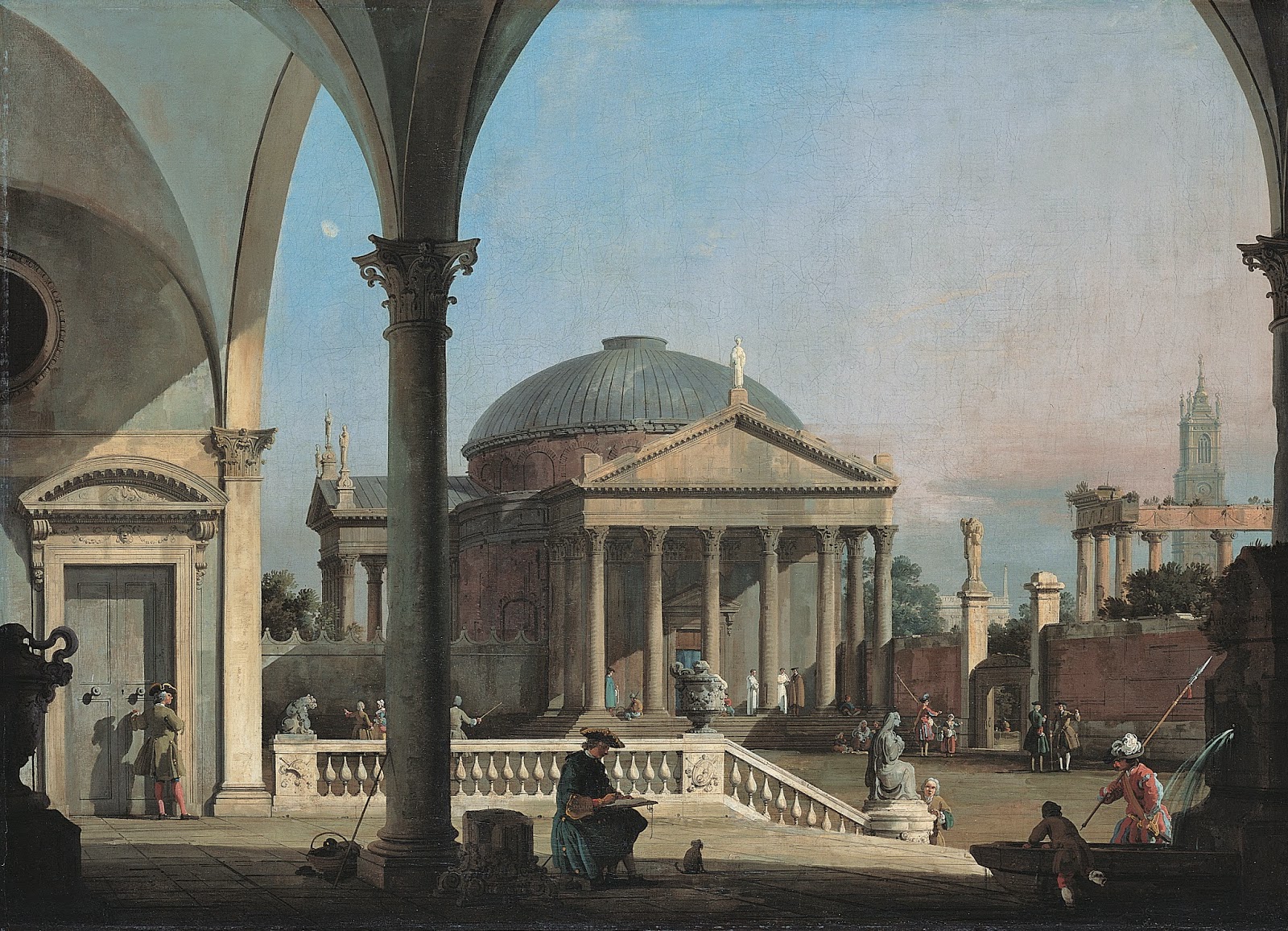The painting, likely from the Renaissance era, depicts a bustling town center under a clear blue sky with some gray clouds. Dominating the scene is an opulent building with tall, elegant stone pillars and a distinctive green domed roof adorned with vertical lines. The architecture, reminiscent of classical Roman style with Greek columns, suggests a highly civilized setting. In the spacious courtyard, people dressed in Revolutionary War-era clothing, including men in knickers and women in long gowns with fancy hats, are engaged in various activities—conversing, writing, and walking. Numerous statues populate the scene, adding to the grandeur and historical richness of the town. The overall ambiance captures a vibrant and structured society deeply rooted in classical architectural beauty.